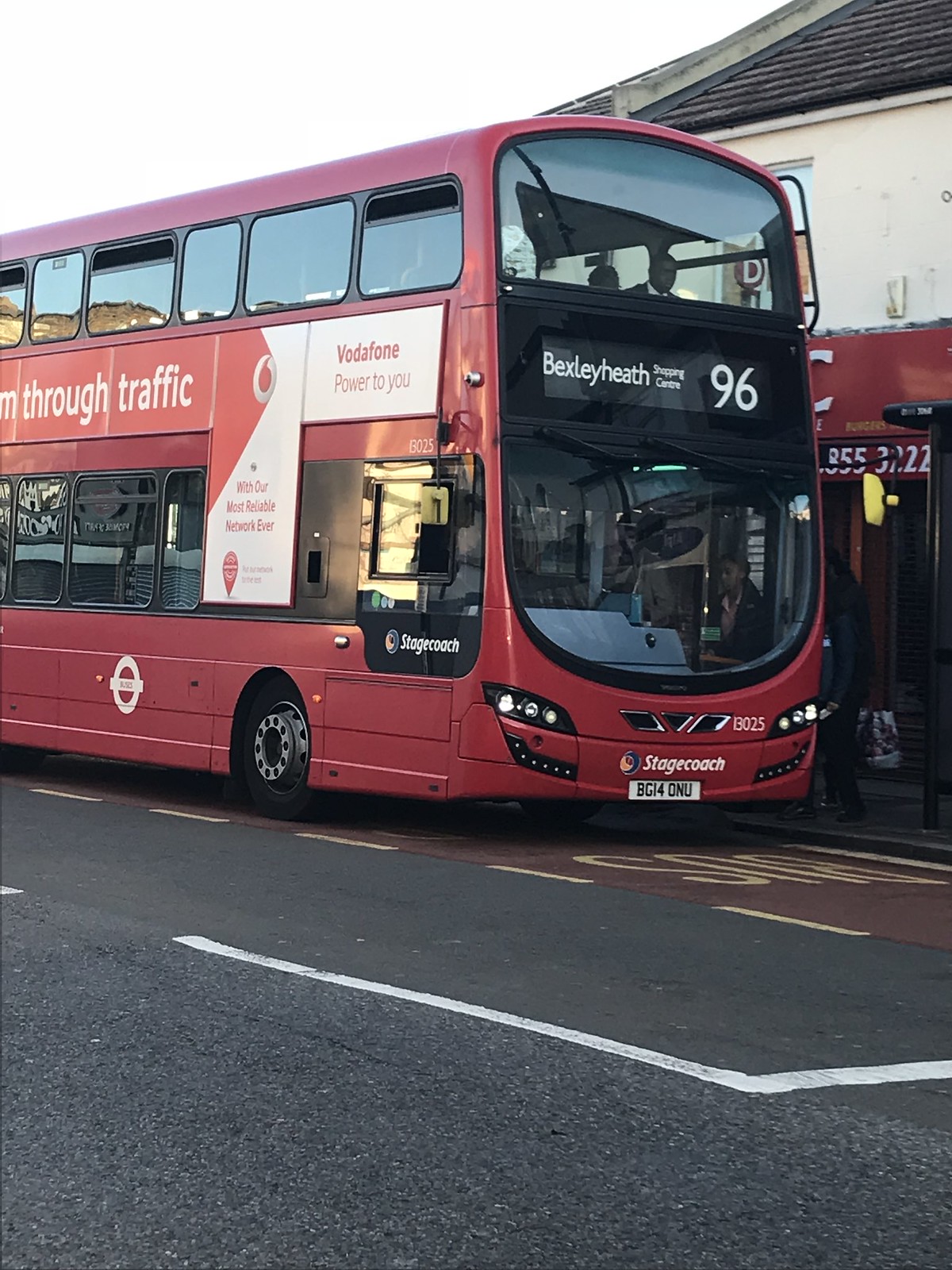The image depicts a photorealistic red double-decker bus prominently positioned just right of center, extending out of the left side of the frame. The bus, facing three-quarters towards the viewer and slightly to the right, features black trim around its windows. The destination marquee on the front reads "Bexley Heath" with the route number "96" clearly displayed to its right. Below the windshield, the word "Stagecoach" is visible, and the bus bears the identification number 13025 as well as a white license plate that reads "BGI40NU."

A yellow side mirror is visible on the bus's right side. The bus lane it occupies is tinged brown with yellow writing, whereas the adjacent road is gray, marked with white lines. On the side of the bus, there are several advertisements, including a prominent red and white sign, and a Vodafone ad proclaiming, "Vodafone power to you with our most reliable network ever." The driver's compartment is discernible, with a driver visible.

The backdrop features a two-story building with a brown exterior and a dark roof, partially obscured by the bus. This building has a red sign with white letters and numbers, possibly reading "855-322." The sky appears white, providing a stark contrast to the colorful elements in the image.